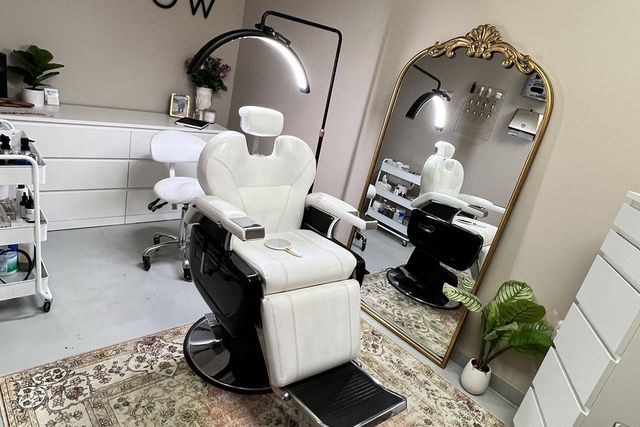This image depicts an upscale hair salon, meticulously designed with a predominantly black and white color scheme. Central to the room is a black and white barber's chair, positioned atop a decorative, cream-colored oriental rug with brownish tones. An antique gold-framed mirror, adorned with ornate designs at the top, leans against the wall, reflecting the chair and adding to the elegant atmosphere. Above the chair, a bright LED light illuminates the space.

To the right, a white, multi-drawer cabinet stands, featuring drawers of different shapes and sizes. Adjacent to the cabinet, a green plant in a white planter adds a touch of nature to the monochromatic decor. The back wall is painted in a subtle beige, with visible trim along the bottom, complementing the plain gray flooring that lies beneath the rug.

On the left side of the room, a white desk adorned with plants and a couple of pictures sits, contributing to the serene and stylish ambiance. A three-tiered cart filled with various salon supplies is also present, indicating the functional aspect of the space. Lastly, a white rolling desk chair is seen in the background, completing the setup of this sophisticated and well-equipped salon.